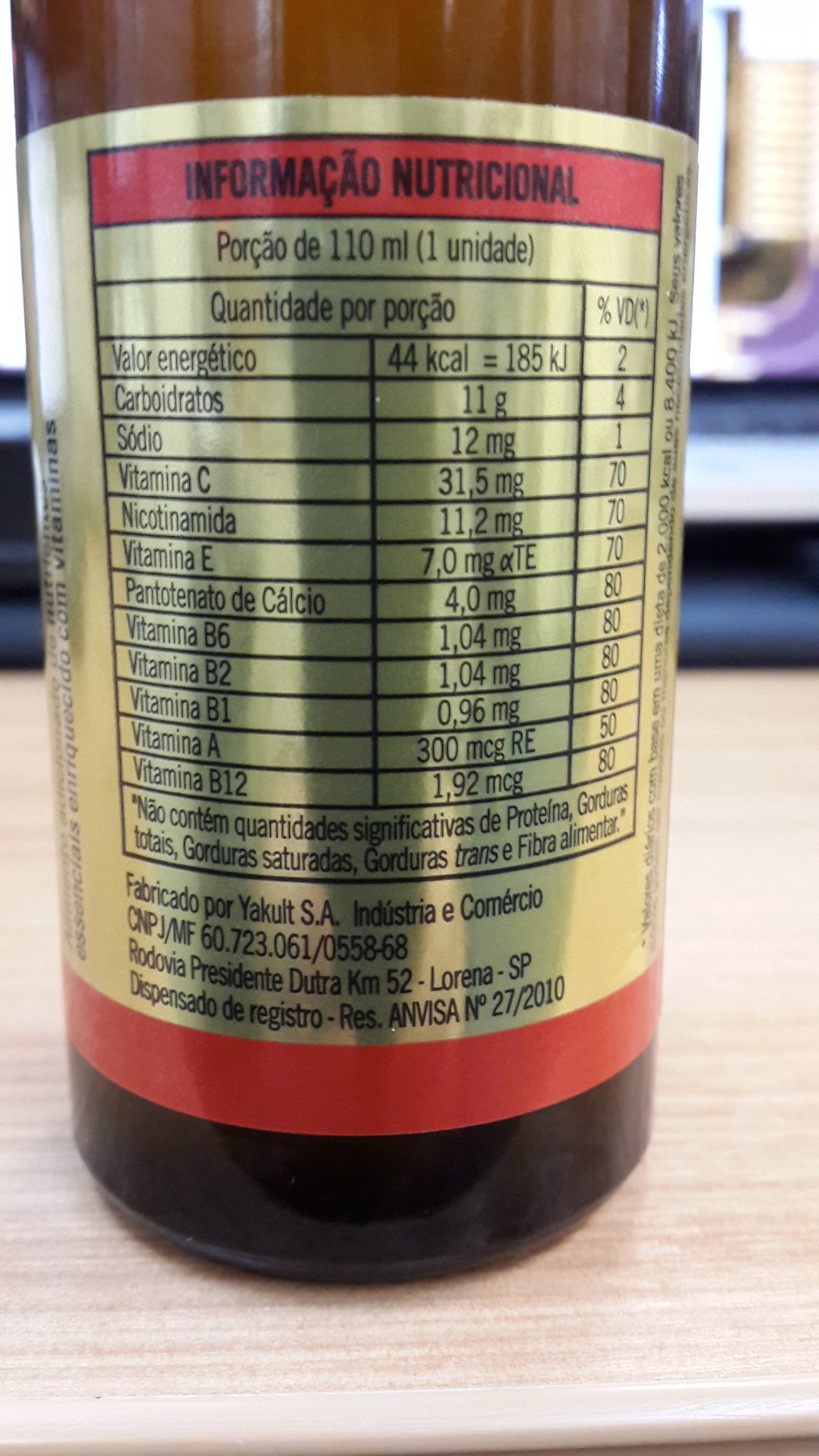A dark amber glass bottle is placed on a light wood surface, capturing the interplay of textures and colors. The bottle exudes an old-world charm with a gold label adorned with red accents and intricate black writing, lending it a touch of elegance. A prominent red stripe encircles the bottle, providing a striking contrast against the dark amber glass. Reflective highlights dance across the top and bottom parts of the bottle, accentuating its glossy finish. The label features nutritional information written in Spanish, showcasing numbers and data that hint at the bottle's contents. Despite the language barrier, the meticulous detail in the bottle’s presentation tells its own compelling story.